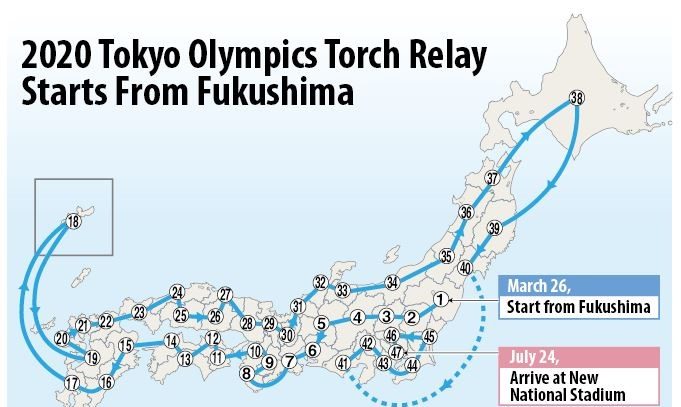This graphic illustrates the 2020 Tokyo Olympics torch relay route across Japan. At the top of the map, the title reads, "2020 Tokyo Olympics Torch Relay." The relay begins on March 26th in Fukushima, marked as number 1 on the map, and progresses through various numbered points connected by a blue line, which winds through Japan's islands. Each marker along the route includes a date, culminating in the final destination, marked as 47, where the torch is scheduled to arrive at the New National Stadium in Tokyo on July 24th. The map effectively visualizes the relay’s extensive pathway, showcasing the journey from start to finish.